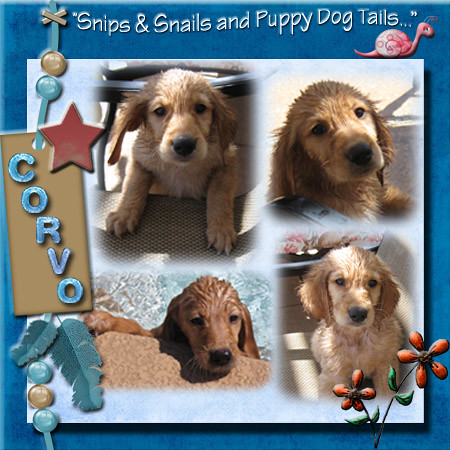The poster is a square with a dark blue background and features a white inner square at the center containing four images of a puppy dog with frizzy, brownish hair, possibly a golden retriever or yellow lab. The top of the poster has white, curved text that reads "Snips and Snails and Puppy Dog Tails..." with a small, pink cartoon snail right below it. On the left side of the poster, the name "Corvo" is spelled out in slanted blue letters within a gold rectangle bordered by a red star and blue leaves, giving it an anime or cartoon-like appearance. The four puppy photos show the dog from different angles: the top left image has the puppy looking straight at the camera with its paws on a table, the top right image shows the puppy's head tilted slightly to the side, the bottom left image captures the dog with its front leg up on the side of what looks like a pool, and the bottom right image features the puppy sitting and staring wistfully ahead. In the bottom right corner, there is a decorative element that resembles a flower stem with red petals.